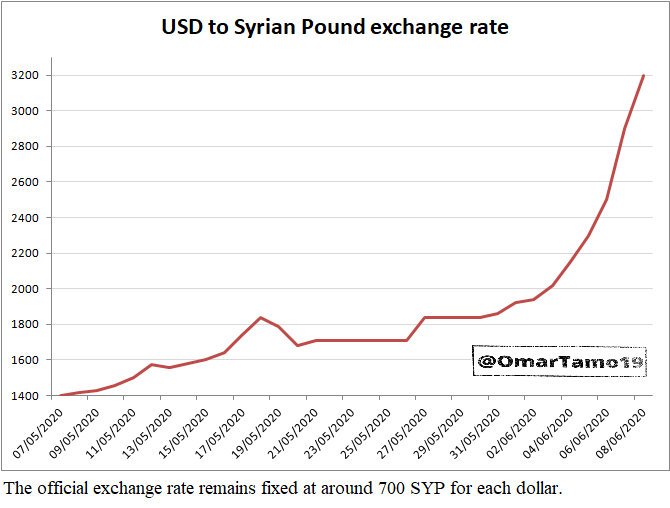This detailed line graph depicts the exchange rate of US Dollars (USD) to Syrian Pounds (SYP) over a time period ranging from May 7, 2020, to June 8, 2020. The title "USD to Syrian Pound Exchange Rate" is prominently displayed at the top center of the graph. The y-axis, though unlabeled, tracks the exchange rate numbers starting from 1,400 up to 3,200 SYP per USD. The x-axis labels the dates in the day-month-year format. 

Initially, on May 7, 2020, the exchange rate is recorded at the baseline value of 1,400 SYP per USD. The red line on the graph shows a gradual increase in the exchange rate with minor fluctuations, reflecting overall upward movement. A significant spike is observed towards the end of the period; between June 6, 2020, and June 8, 2020, the rate escalates sharply from around 2,000 to 3,200 SYP per USD. This increase highlights the currency's depreciation during the mentioned period, possibly influenced by the COVID-19 pandemic.

At the bottom of the graph, it mentions that the official exchange rate remains fixed at approximately 700 SYP per USD, which contrasts sharply with the market rate depicted. Additionally, a watermark labeled "@OmarTamo19" suggests ownership or authorship of the graph.